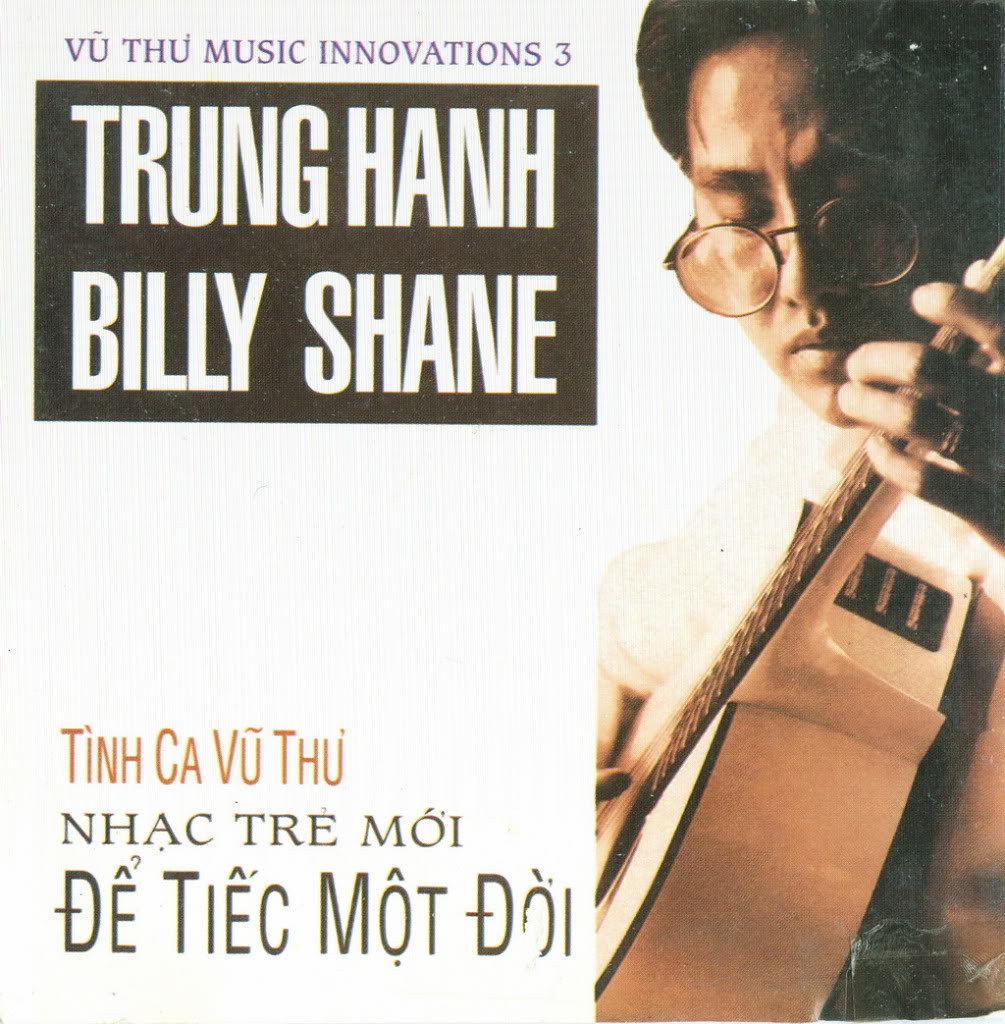A vintage-style advertisement possibly from the 1980s showcases Vu Thu Music Innovations 3. The poster features a man with round eyeglasses playing a distinctive white acoustic guitar on the right-hand side, exuding a classic 80s vibe. On the left side, the headline prominently reads "Vu Thu Music Innovations 3," followed by the names "Trang Han" and "Billy Shane." In the lower left corner, the name "Tin Ka Vu Thu" is visible, accompanied by additional text in a foreign language, adding to the nostalgic feel of the advertisement. The overall design appears aged and dated, reminiscent of the advertising style from a few decades ago.